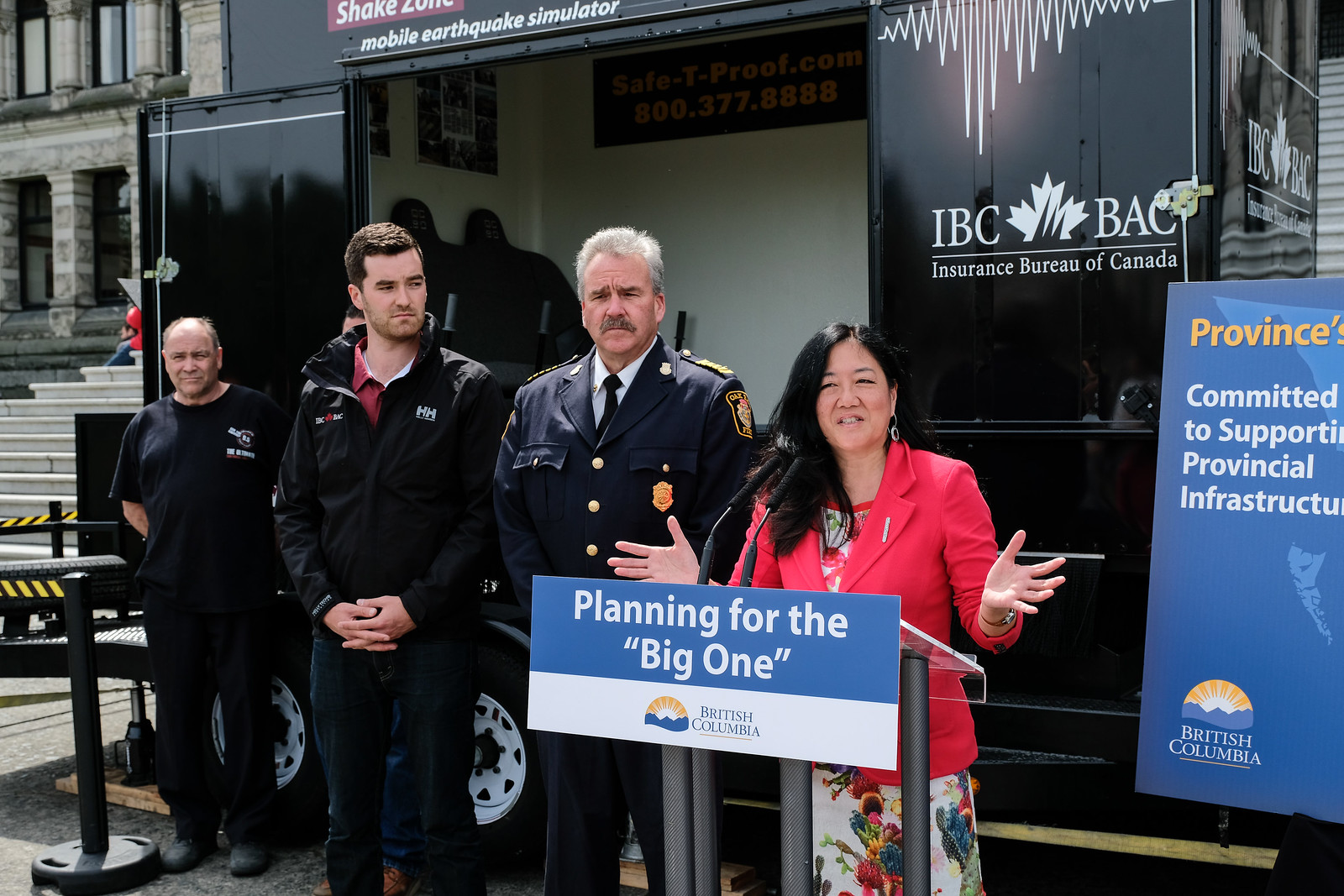In the image, an Asian woman with long dark hair stands poised at a clear podium with gray posts, delivering a speech. She is elegantly dressed in a white dress adorned with a vibrant floral design featuring colors such as red, orange, blue, green, and yellow. Over her dress, she wears a red blazer jacket. The podium displays a sign that reads "Planning for the Big One, British Columbia," accompanied by a yellow sun symbol above blue waves. 

To her left stands a white police officer or sergeant, characterized by his gray hair and thick mustache, dressed in a blue uniform with silver and gold badges. Next to him, another white male can be seen wearing a red polo shirt covered by a black windbreaker jacket and blue jeans. Further to their left is another man, possibly Latino, dressed in black. A fourth individual, partially visible, appears to be wearing an all-black outfit.

Behind the group, a large black bus is visible, bearing the inscription "IBC BAC, Insurance Bureau of Canada." The bus is part of the "Shake Zone" mobile earthquake simulator, as indicated by additional signage. On the woman's left, there is a blue sign with yellow and white text that highlights provincial commitments to infrastructure support, further emphasizing the setting in British Columbia.